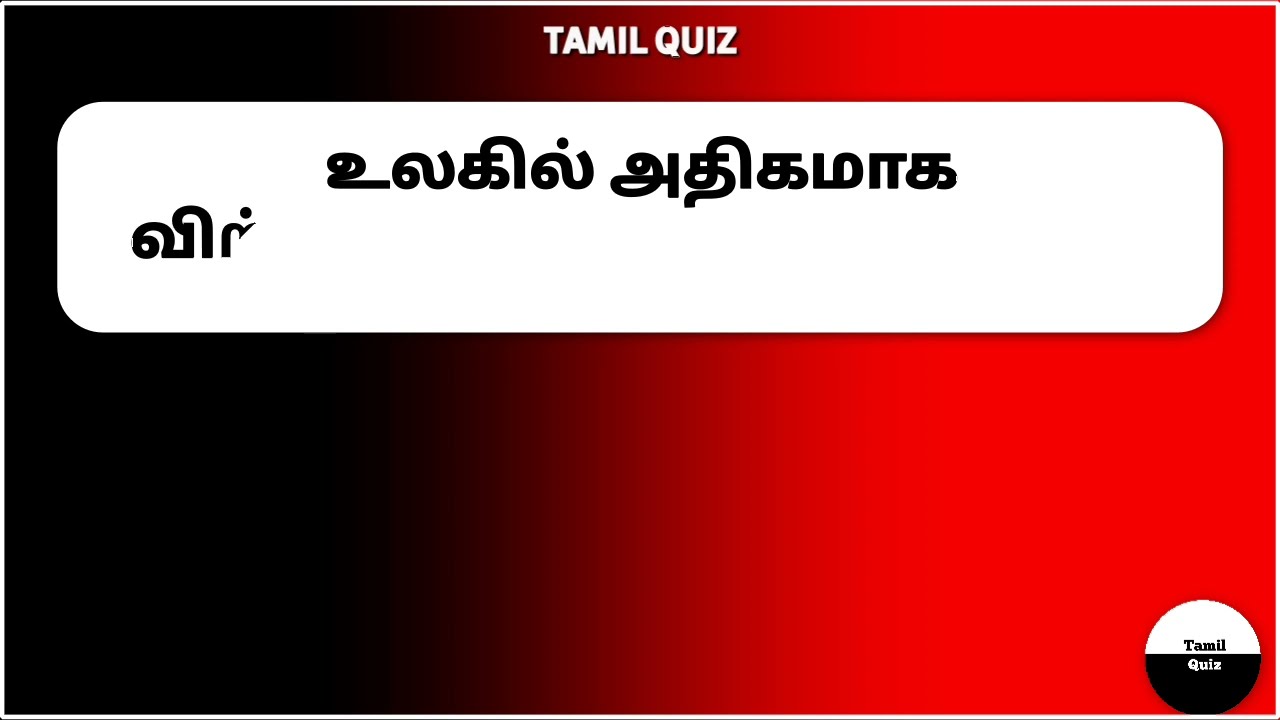The image depicts a slide for a presentation designed as a quiz. The background of the slide transitions from black on the left to red on the right, creating a striking gradient effect. At the top of the slide, there is a prominent white rectangle with curved corners, featuring black text written in an unfamiliar script, likely an Indian language. Above this white rectangle, the title "Tamil Quiz" is written in white text. In the lower right corner of the slide, there is a distinctive circle, split into two halves: the top half is white with the word "Tamil" in black print, and the bottom half is black with the word "Quiz" in white print.